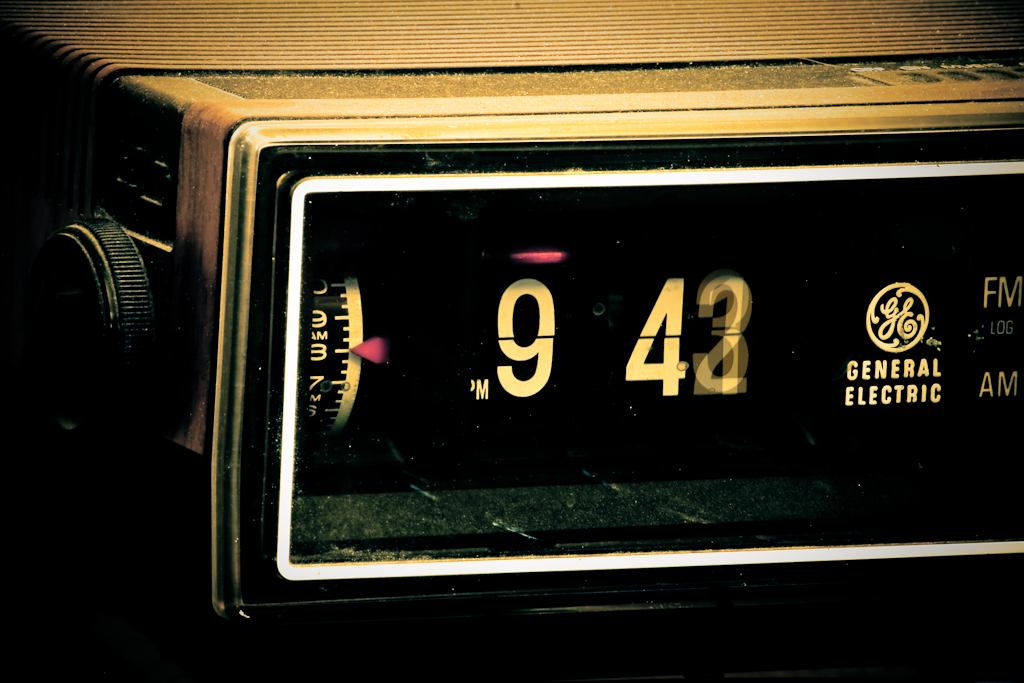A vintage digital alarm clock with a distinct 80s to mid-90s design is the focal point of this image. The clock displays the time as 9:43 PM, captured with a subtle blur on the digit '3', suggesting the moment it transitioned from '2' to '3'. The display features classic rolling plastic numbers, typical of the era's technology. To the left side of the clock, a radio tuning knob is visible, emphasizing the clock's dual functionality as both a timekeeper and a radio. The nostalgic aesthetic of the clock is accentuated by its retro design elements, evoking memories of a bygone era.